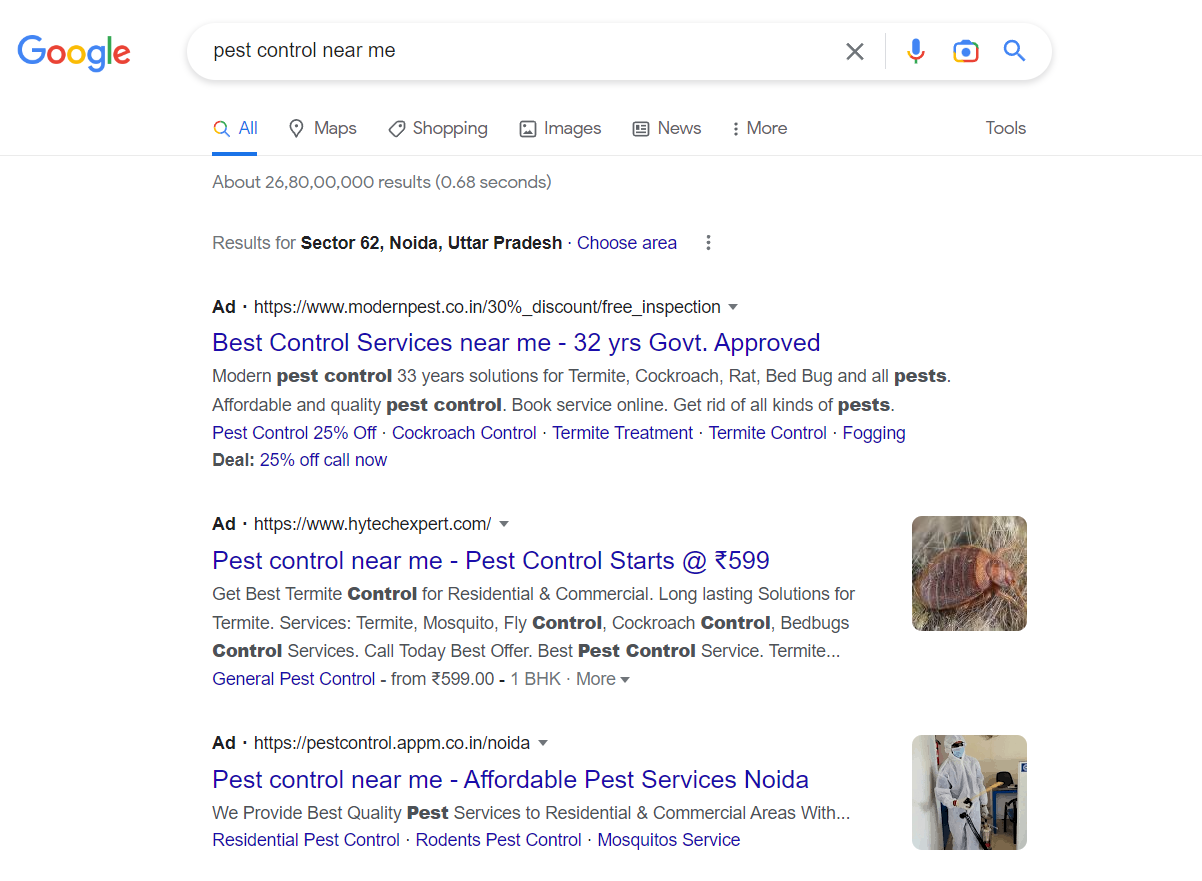A screenshot of a search engine results page reveals the following: 

**At the top**, the Google logo appears with the letters: "G" (blue), "o" (red), "o" (yellow), "g" (blue), "l" (green), and "e" (red). Below this, a search bar contains the query "Ovilus pest control near me". Icons for a microphone (voice search), camera (image search), and magnifying glass (search) are visible.

**Below the search bar**, navigation tabs include "All", "Maps", "Shopping", "Images", "News", and "More Tools". The search results indicate approximately 26.8 billion results retrieved in 0.68 seconds.

**Highlighted Results for 'Sector 62'** include several websites and snippets:
1. **Modern Pest Control Services** - A listing mentions services in Sector 62 with 30 years of experience. They offer solutions for termites, cockroaches, rats, bed bugs, and other pests. Services are described as affordable and of high quality. Promotions include a 30% discount and a free inspection, with the company being government-approved.

2. **HiTech Expert Pest Control** - This site offers pest control for both residential and commercial properties. Services cover termites, mosquitoes, flies, cockroaches, and bed bugs. There is a mention of a comprehensive treatment for termites at a cost of ₹599.

3. The link **"https://pestcontrol.appio.co.in"** also pops up, promising affordable pest control services.

The search results collectively emphasize various pest control services with offers for online booking, discounts, and long-lasting solutions. Central themes include termite treatment, cockroach control, fogging services, and a general pitch for quality pest management at competitive prices.